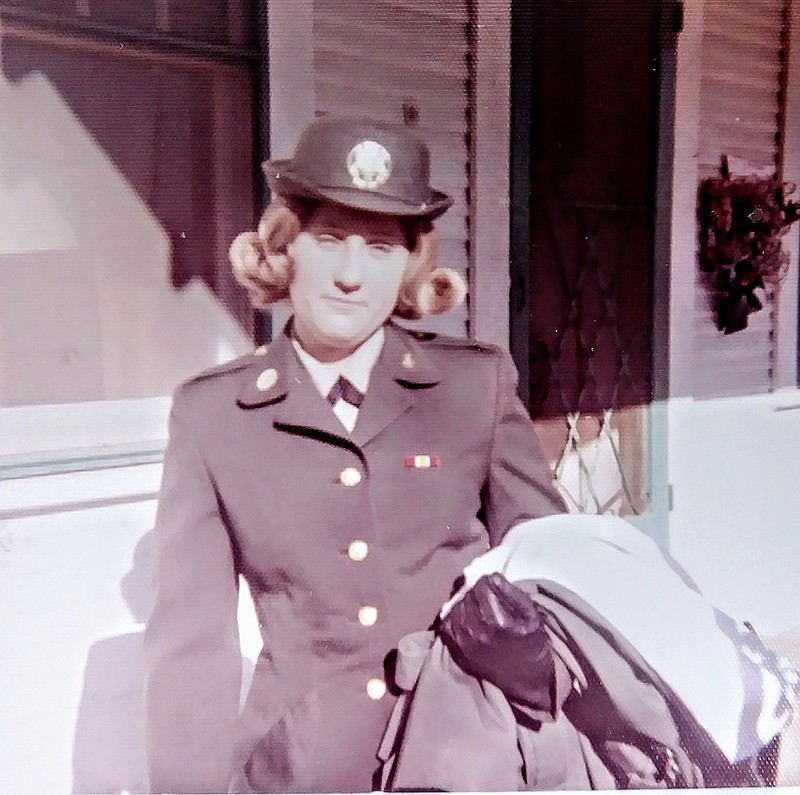The image features a photorealistic, vintage-style photograph of a white woman in a formal uniform, indicative of either a police officer or a member of the Women's Army Corps, likely from the 1940s to 1980s. She is sporting a stern, unsmiling expression and has short, curled brunette hair that almost touches her shoulders. Atop her head is a black hat adorned with an emblem or badge at the center. Her uniform is meticulously detailed, featuring a crisp white shirt, possibly with a blue collared tie, and a jacket fastened with four large gold buttons and additional buttons at the lapels. Her left hand, clad in a black glove, holds a pile of garments or a longer coat draped over her forearm. The setting is in front of a house with white siding, a black door positioned to her right, and a window with floral decorations to her left. Additionally, the door has a sack for holding mail and the elements suggest a mid-20th-century residential background.